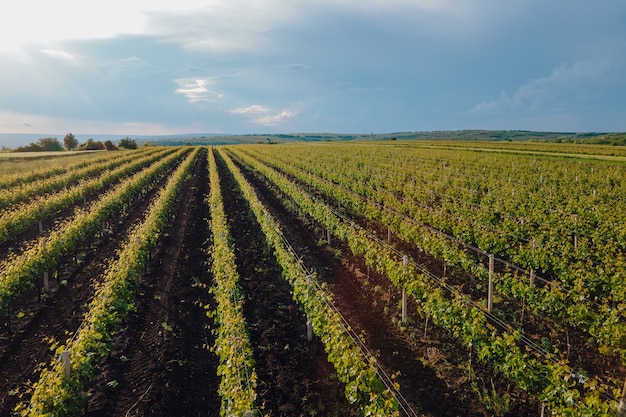The photograph captures a vast, meticulously cultivated farm field extending into the distance, featuring neat, evenly spaced rows of deep lush green plants. The plants, possibly soybeans or grapevines, are supported by trellises to prevent them from falling over. The rows start wider in the foreground and narrow as they recede towards the horizon, giving a sense of great depth and size, potentially spanning up to a mile. The plants boast multiple flowery leaves atop them, and the space between the rows is filled with rich brown soil, suggesting they might still have some growing to do. The sky above is a striking deep blue adorned with wisps of white, pillowy clouds, adding a sense of serene beauty to the expansive landscape. In the background to the far left, a small cluster of trees can be seen, while the rest of the image is devoid of people, animals, buildings, or any motorized vehicles, emphasizing the field's sprawling natural tranquility.